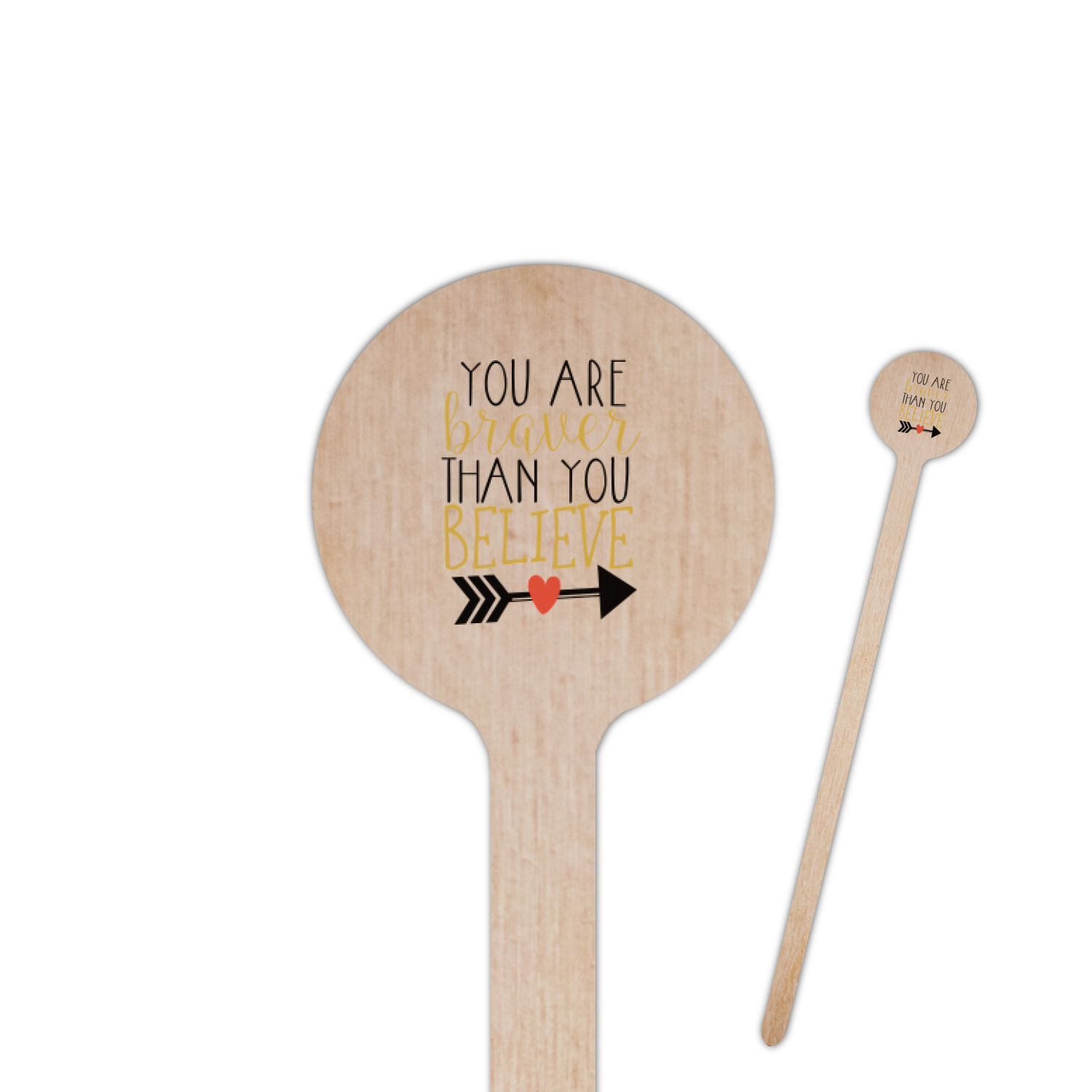The image depicts a light tan wooden sign, resembling a very long balsa wood or popsicle stick stake. At the top of the stake is a small, round sign. The right side of the image shows a smaller version of this sign, providing a full view of the item, while the left side offers a close-up of the round top. The sign bears an inspirational message written in black and yellow or gold font: "You are braver than you believe." The words "You are" and "than you" are in black, while "braver" is in cursive yellow and "believe" is in yellow all caps. Below the text is a decorative black arrow with three chevrons representing feathers at the tail, and a little red heart at the center of the arrow's shaft.